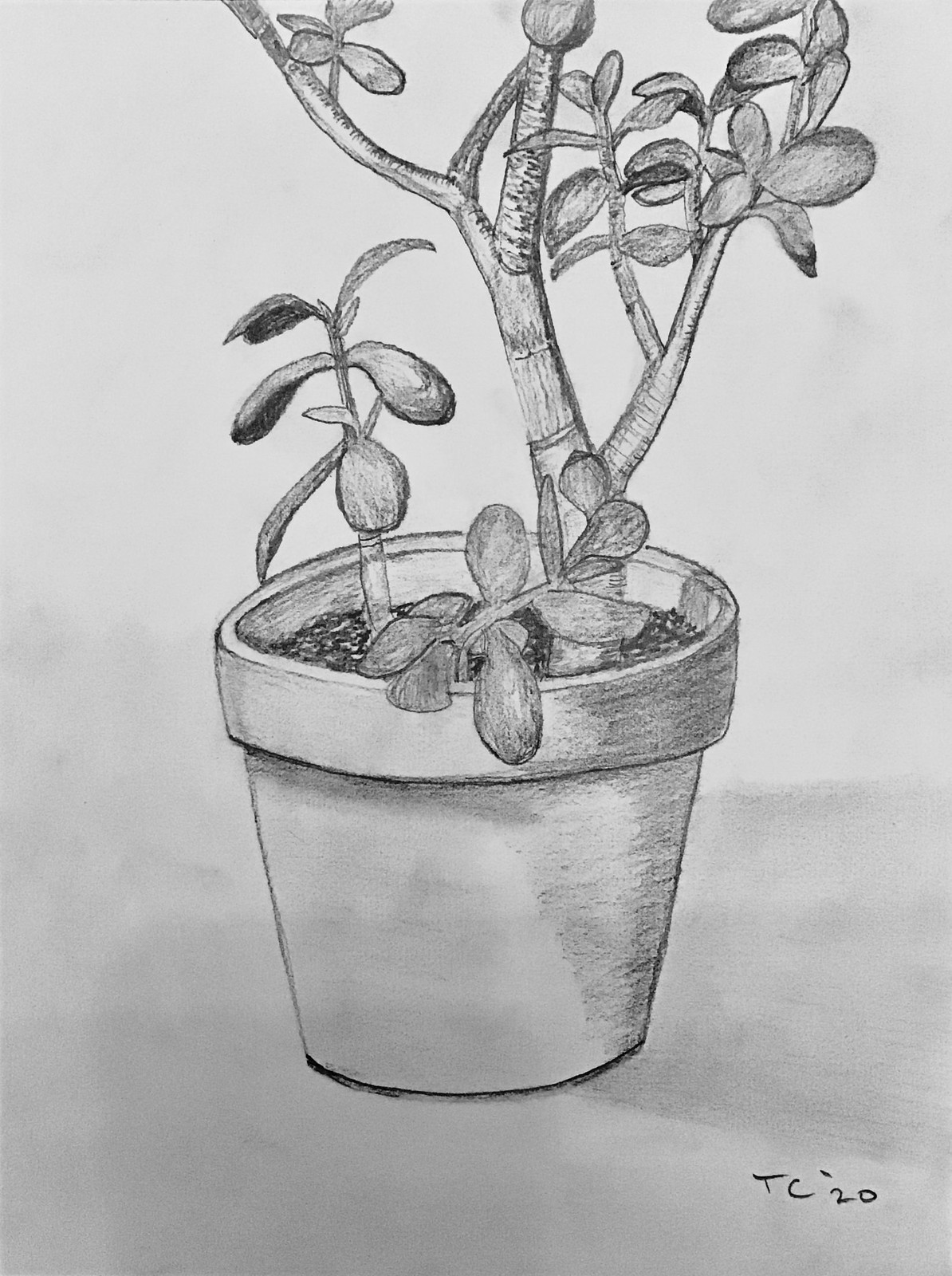The image depicts a black-and-white pencil drawing of a potted plant on sketchpad paper. The plant, reminiscent of a jade plant with its thick stalks and delicate, paddle-shaped leaves resembling raindrops, is housed in a terracotta-type pot. The pot features visible shading on its right side, suggesting a light source from the left. The drawing captures the darkness of the soil and intricate details of the plant's stems and leaves. Notably, the top of the plant is cut off, indicating that the entire plant is not visible within the frame. This artwork, potentially a mixed media piece incorporating both pencil and charcoal, includes a signature in the bottom right corner that reads "TC 20". The overall aesthetic gives a realistic portrayal, emphasizing the contrast between light and shadow.